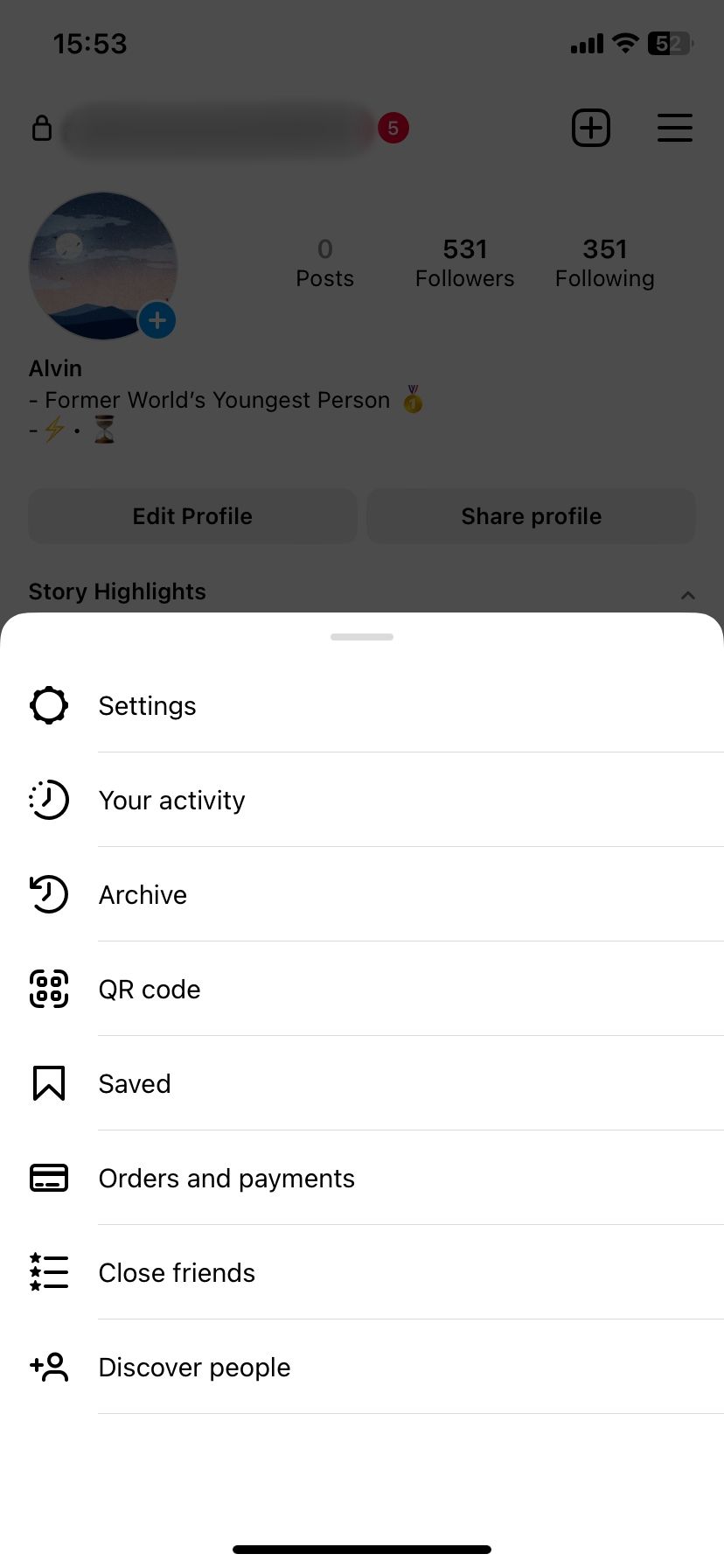This image is a detailed screenshot of an Instagram profile page on a mobile device, showcasing both the standard user interface and a pop-up options menu. 

The topmost section displays the mobile UI elements in black on a white background. The time is indicated as 15:53 on the top left. On the top right, there is a signal strength icon showing four bars, a fully connected Wi-Fi icon, and a horizontal battery icon displaying 52%.

Directly below this section, the foreground includes various UI icons. On the far left is a lock icon, which is followed by a blurred-out section (possibly showing edited or sensitive information). To the right, there's a red symbol, a plus sign, and a hamburger menu (three horizontal lines). 

The profile section of the image has the user's avatar on the left. The avatar seems to depict a sky scene with either a sun or moon, accompanied by clouds and mountain tops. There is a small plus sign overlay at the bottom right of the avatar, typically indicating a story addition option. To the right of the avatar, the profile displays "0 posts," "531 followers," and "351 following."

Under the profile information, there is a description: "Alvin," followed by "Former world's youngest person" with an award emoji. Below this line, an entry reads with lightning bolt and hourglass emojis. The "Edit Profile" button is positioned on the left, while "Share Profile" can be found on the right.

Next, "Story Highlights" is prominently displayed in black text. This is where the pop-up menu begins, covering the lower half of the screen in a white overlay that dimly obscures the background content. The pop-up menu consists of ten selectable options, each accompanied by an icon on the left. The options listed are: Settings, Your activity, Archive, QR code, Saved, Orders and payments, Close friends, and Discover people. These options are separated by thin gray lines for easy navigation.